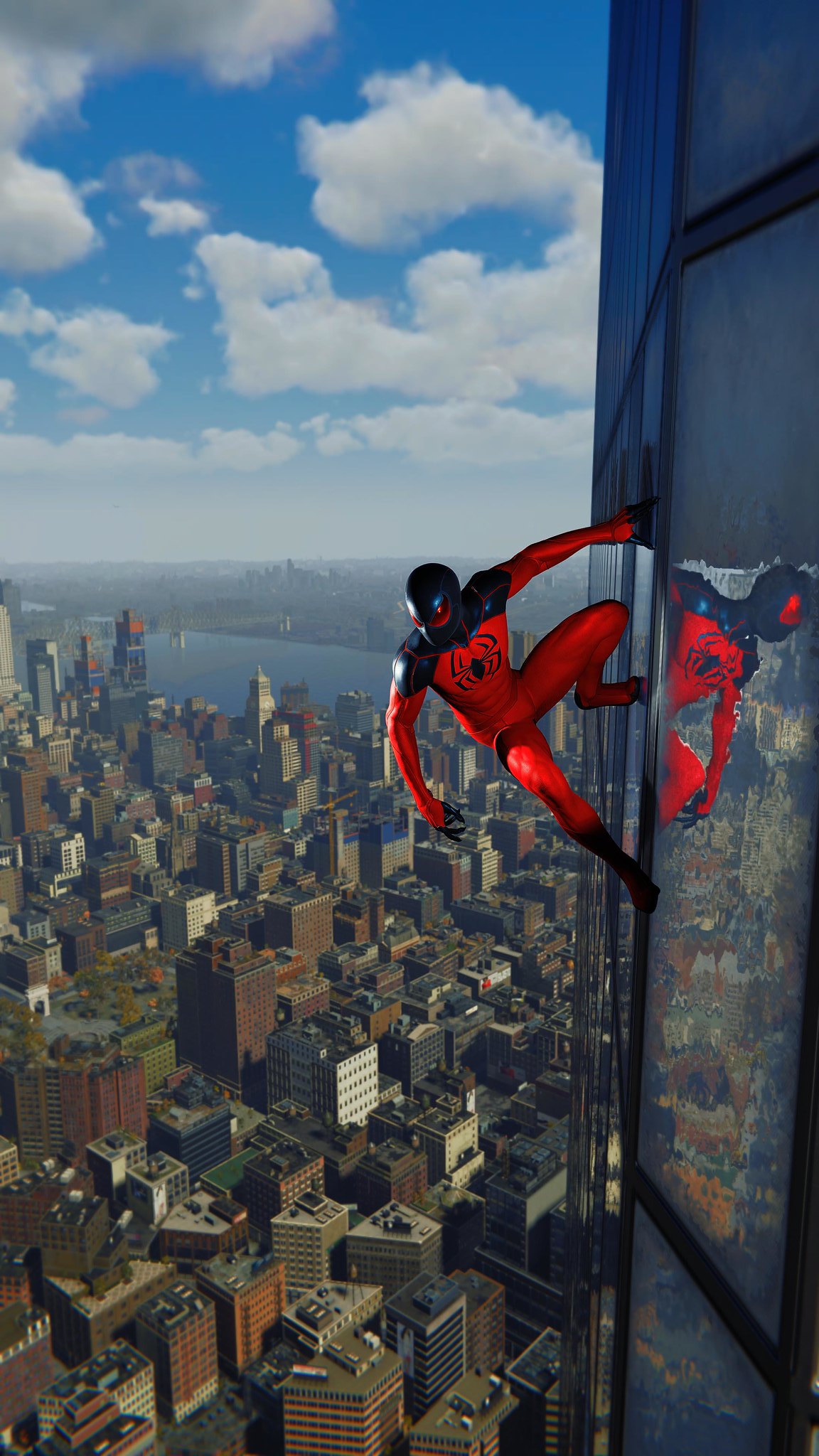In this captivating image, a man dressed in a vibrant red superhero suit with black trim clings dramatically to the side of a tall, glass-paneled building positioned on the right. The superhero, reminiscent of Spider-Man but with a unique costume featuring navy blue shoulders, a black head covering, and a distinctive black spider emblem on his chest, strikes a dynamic pose with one hand and both feet gripping the building. His left hand braces him while his right arm hangs by his side, and his left leg is bent upward in a poised position. The urban backdrop is breathtaking, showcasing a sprawling, colorful cityscape filled with skyscrapers and medium-height buildings extending into the distance. Over the horizon, a river winds through the city, crossed by a bridge, adding depth to the composition. The scene is bathed in brilliant daylight under a bright blue sky dotted with numerous puffy white clouds, enhancing the vibrant and lively atmosphere encapsulated in the image.